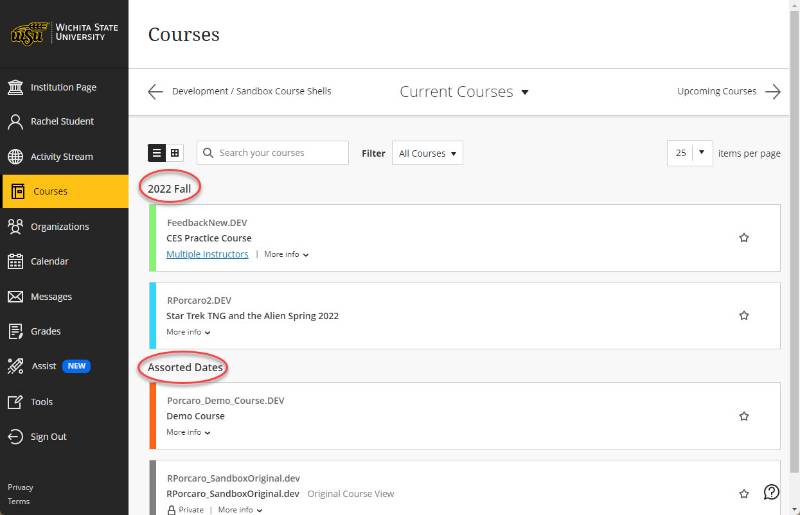This screenshot captures the Wichita State University (WSU) website. The WSU logo is prominently displayed in the top-left corner, embedded within a vertical banner along the left side. The sidebar contains numerous subcategories including Institution Page, Students, Activity Stream, Courses (which is currently selected), Organizations, Calendar, Messages, Grades, Assist, Tools, and a link to Sign Out. Additional links for Privacy and Terms are located at the bottom of the sidebar.

The main page is titled "Courses," displaying various subcategories such as Upcoming Courses and Sandbox Course Shows, which allow navigation through left and right arrows. Under the Current Courses section, entries such as "2022 Fall" and "Assorted Dates" are marked with pinpoints for easy identification. The page itself features a clean, minimalist design with a white and grey color scheme, reflecting an organized and user-friendly layout.